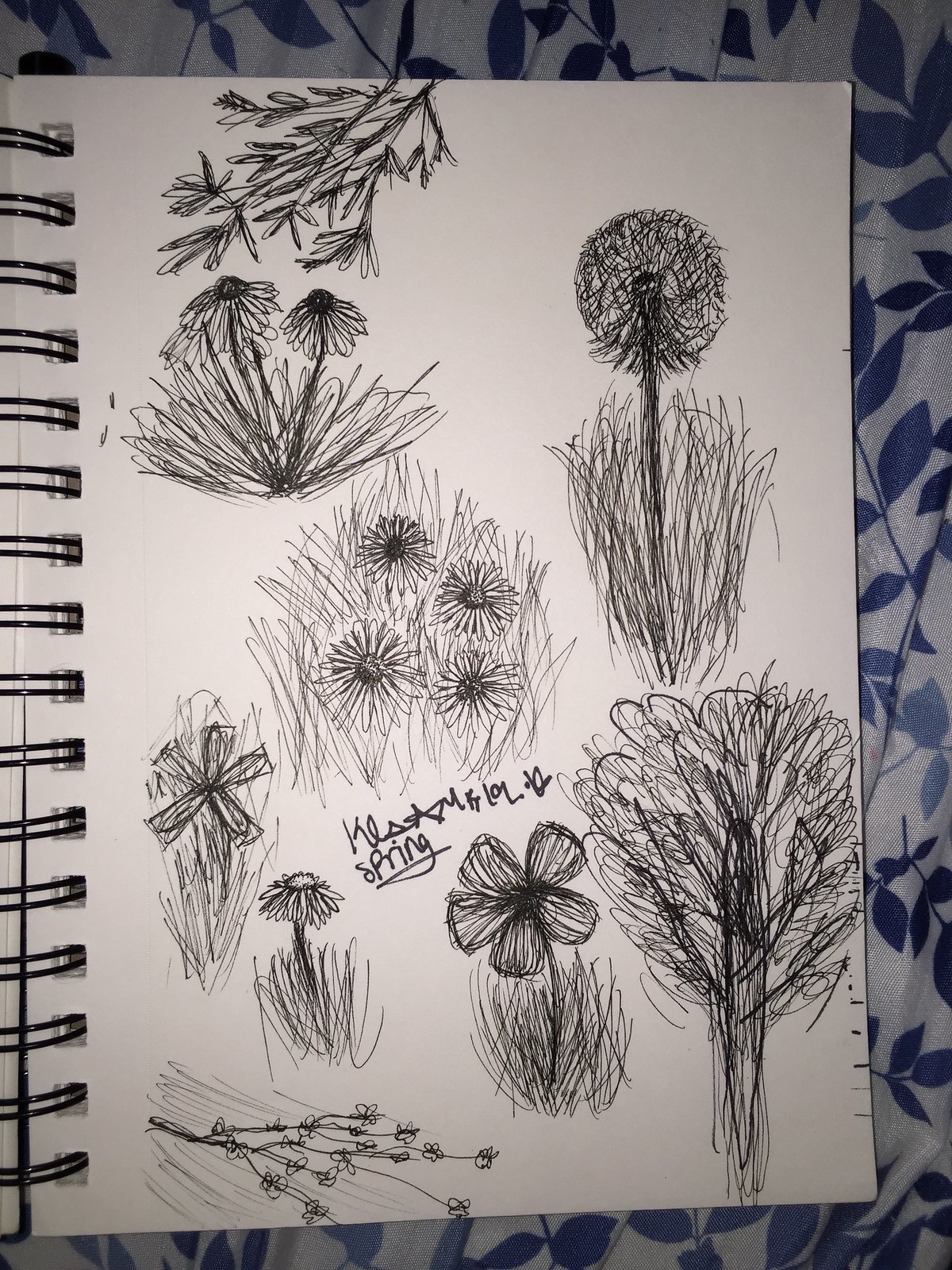This detailed black-and-white sketch, meticulously drawn with pen, is showcased on a white notebook with a black spiral binding. The artwork features an array of botanical elements, highlighted by two prominent daisy-like flowers emerging from a patch of grass. Around them, delicate leaves reminiscent of those from a tree add diversity to the composition. A singular dandelion stands tall, sprouting from its own grassy base, capturing the essence of a breezy spring day. Another flower with distinctive petals makes a unique appearance, although its species remains unidentifiable. The artist has thoughtfully signed her name and inscribed the word "spring," encapsulating the season's vibrant spirit in every stroke.